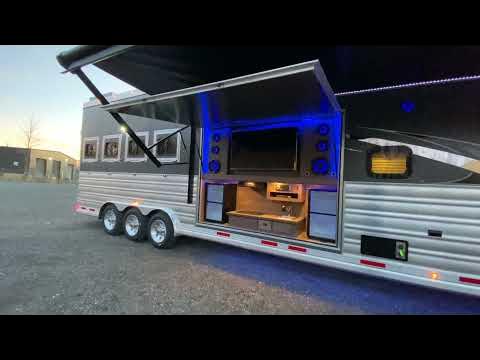The photograph features a sleek, silvery vehicle that could be a luxurious tour bus or an elaborate horse trailer, though its exact purpose remains ambiguous. The vehicle is angled away from the viewer, with its rear pointing towards the upper left-hand corner of the image. It's equipped with three wheels in a row on its rear section, indicating a substantial and possibly heavy structure.

Dominating the foreground, the vehicle's side features an open hatch, revealing a compartment illuminated with blue lighting. Inside this compartment, there are two sets of drawers or possibly speakers, along with a small platform, suggesting some sort of storage or entertainment functionality. Above this open hatch, a mounted screen—possibly a computer or television—is flanked by three speakers on each side, all lit by the blue lights.

The rear of the vehicle has four windows positioned above the triple-wheel setup, reinforcing the idea that it is built to carry considerable weight. Atop the entire structure, a removable canopy, which could serve as protection against rain or sun, is visible.

In the distant background, a hazy blue sky, a tree, and a structure with three large garage doors can be seen. The paved ground in the foreground underscores the vehicle as the central focus of the photograph. The overall scene exudes a sense of modernity and purpose, even if its exact function is not immediately clear.